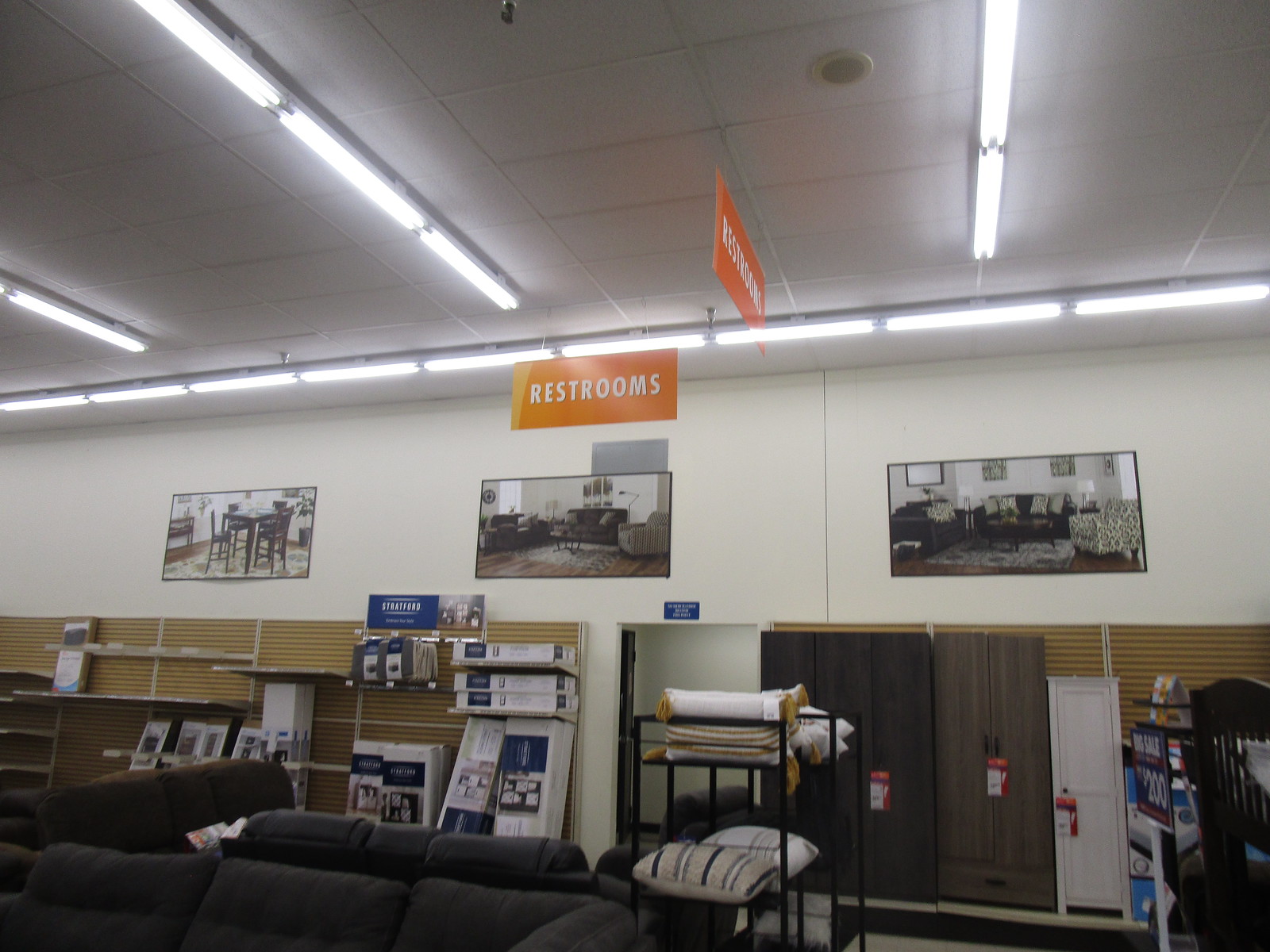The photograph, taken in landscape orientation, captures the interior of a store. The central focus is a back wall framed by an industrial ceiling that occupies the top third of the image. This ceiling features a rectangular acoustic panel and is lined with both a rear row and three perpendicular rows of thin, bright fluorescent lights, creating a stark illumination.

At the upper back of the image, an orange rectangular sign with white text marks the location of the restrooms. Below this sign, the back wall is adorned with three large photographs: the left photograph showcases a dining room table surrounded by chairs, while the center and right photographs highlight living room arrangements with couches, chairs, and rugs, all depicted in black and white. 

The wall also features several shelves, filled with boxed items and what appear to be tabletops stored flat. A small blue sign is positioned above an opening between two shelves in the middle of the wall. In the bottom left corner of the image, the edge of a couch is visible on the floor, suggesting the space is part of a furniture store showcasing its products.